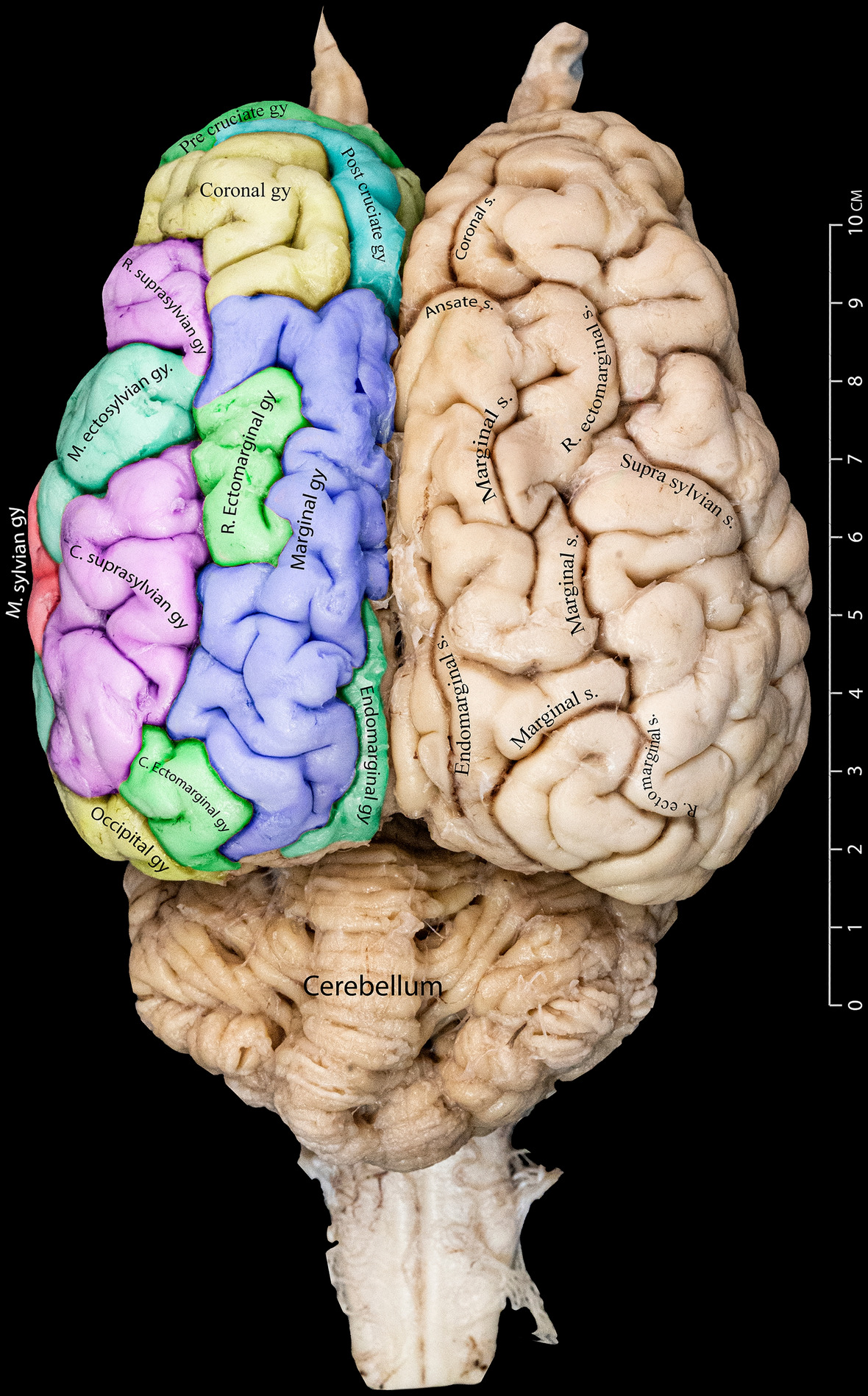The image displays a detailed diagram of a brain with a clear division between the left and right hemispheres. The right hemisphere is depicted in natural colors, highlighting the white matter and intricate gyri typical of a brain's appearance, while the left hemisphere is color-coded in shades of blue, green, purple, and yellow to differentiate the various sections, each labeled with specific anatomical names such as Marginal S, Suprasylvian R, and Ectomarginal. Both hemispheres, though differing in color representation, feature comprehensive labeling that includes the cerebellum and brainstem, which extend downward from the main brain mass. The cerebellum appears as a singular piece with distinct lines and remains in a natural tan color. Adjacent to the brain image, on a black background, is a white centimeter ruler ranging from 0 to 10 cm, providing a scale for the brain's size from the base to the top.